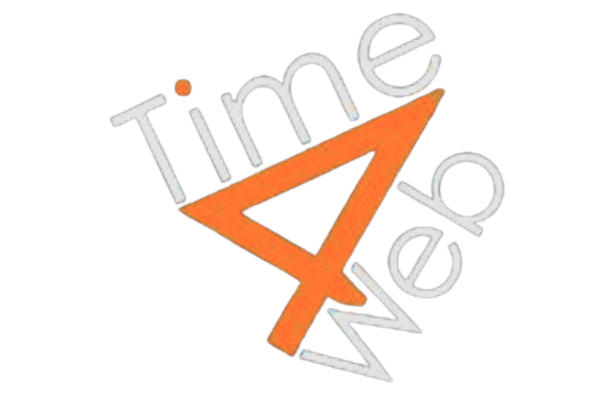The image is a PNG with a clear white background, prominently featuring a logo consisting of the word "time," the number "4," and the word "web." The word "time" is written in light gray font with a dark gray outline, slanting upward at about a 30 to 45-degree angle. Notably, the dot on the 'i' in "time" is orange. The orange number "4" is centrally positioned in the image, tilted slightly, with the long edge of the "4" aligned with the upward diagonal of "time." The bottom protruding part of the "4" nestles perfectly within the second peak of the "W" in "web," effectively connecting the two words. The word "web" is also in light gray with a dark gray outline, slanting similarly upward to the right. The cohesive design and color scheme suggest that this image is a well-thought-out logo or brand label.